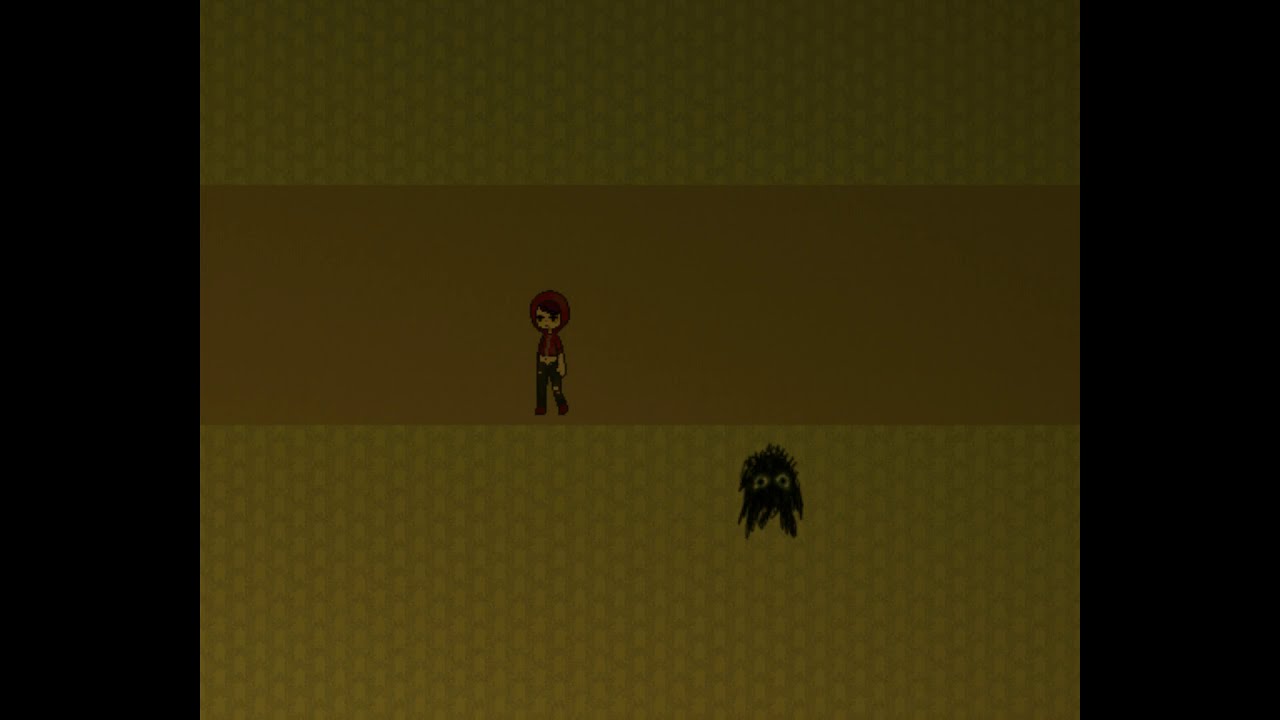The image is a screenshot of a low-pixel video game interface divided into three horizontal sections. The top and bottom sections are yellow with small, rectangular patterns that resemble a computerized grain field or honeycomb texture. The middle section, which is darker in color, varying between brown and olive green, features a cartoon girl standing in its center. She wears a pink headband, a red cropped hoodie revealing part of her stomach, and blue jeans. The girl is staring straight ahead. Thick black borders run along the left and right sides of the image. Near the bottom yellow section, there is a black, ghost-like face with straight-up hair, big eyes that are alternately described as yellow, greenish, or white, adding an eerie element to the scene.